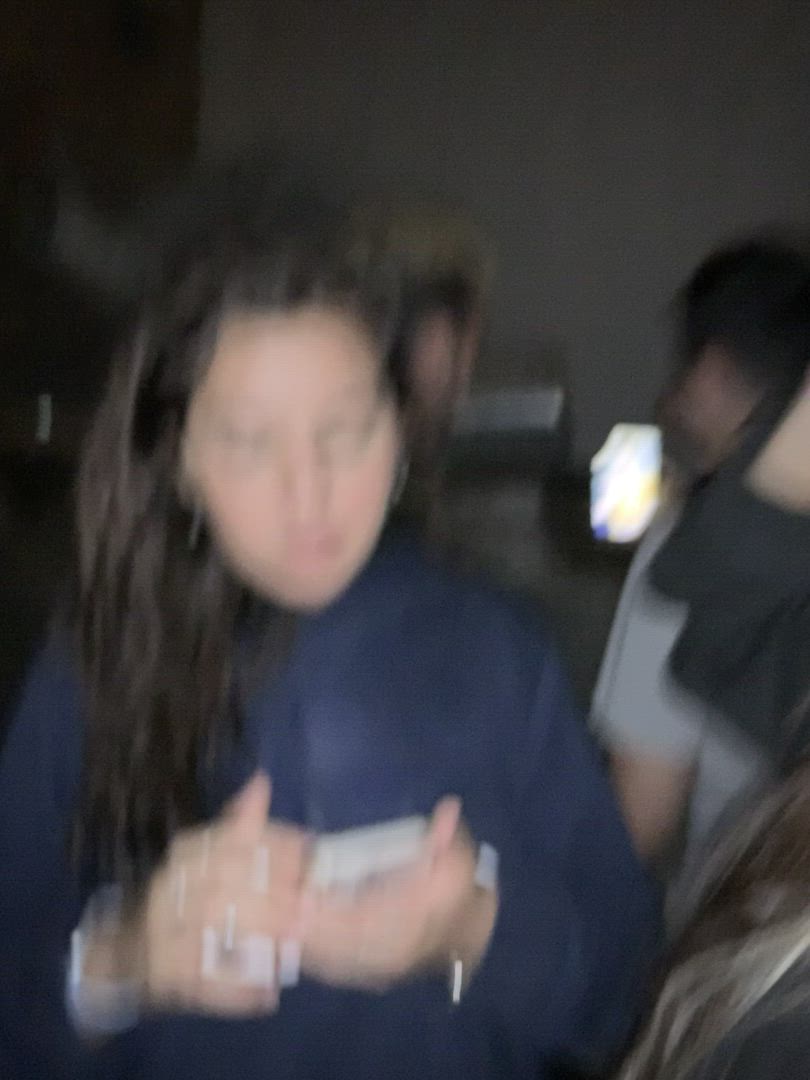The blurry image captures a girl with long brown hair pushed to the side, focused intently on a cell phone she is holding with both hands. She is dressed in a high-collared black jacket and appears to have earrings. Her left hand supports the phone, while her right hand interacts with its screen. She is situated in a room with other people; one is behind her, possibly a bearded man with sideburns, and another to her right, dressed in a short-sleeved white t-shirt beneath a dark silhouette that might be a woman with a black pocketbook. The light in the room casts a dim glow, illuminating the varied brown materials in the lower right of the image. Her skin is pale, and the top of her phone is white, contrasting with its bright screen. In the background, there's another person with short hair, wearing a gray t-shirt and seemingly engrossed in their own cell phone, which displays a burst of colorful light.